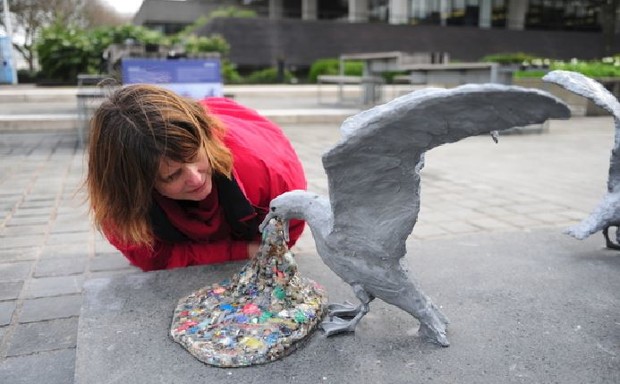In the center of an office building courtyard filled with muted grays, a woman with shoulder-length brown hair intently examines a concrete-like sculpture. She is bent over, wearing a reddish jacket. The focal point of her attention is a detailed sculpture of a gray seagull, positioned with its wings raised in a V shape. The seagull's mouth is open, facing downward, as it appears to vomit a colorful, resin-like material composed of reds, blues, greens, whites, blacks, and grays. This vivid, blobby substance spews out onto a low concrete slab, resembling either trash or other debris. Nearby, part of another seagull sculpture is partially visible, showing only a tail and wing. The woman’s expression suggests a mixture of curiosity and disgust as she closely inspects the seagull's bizarre display.